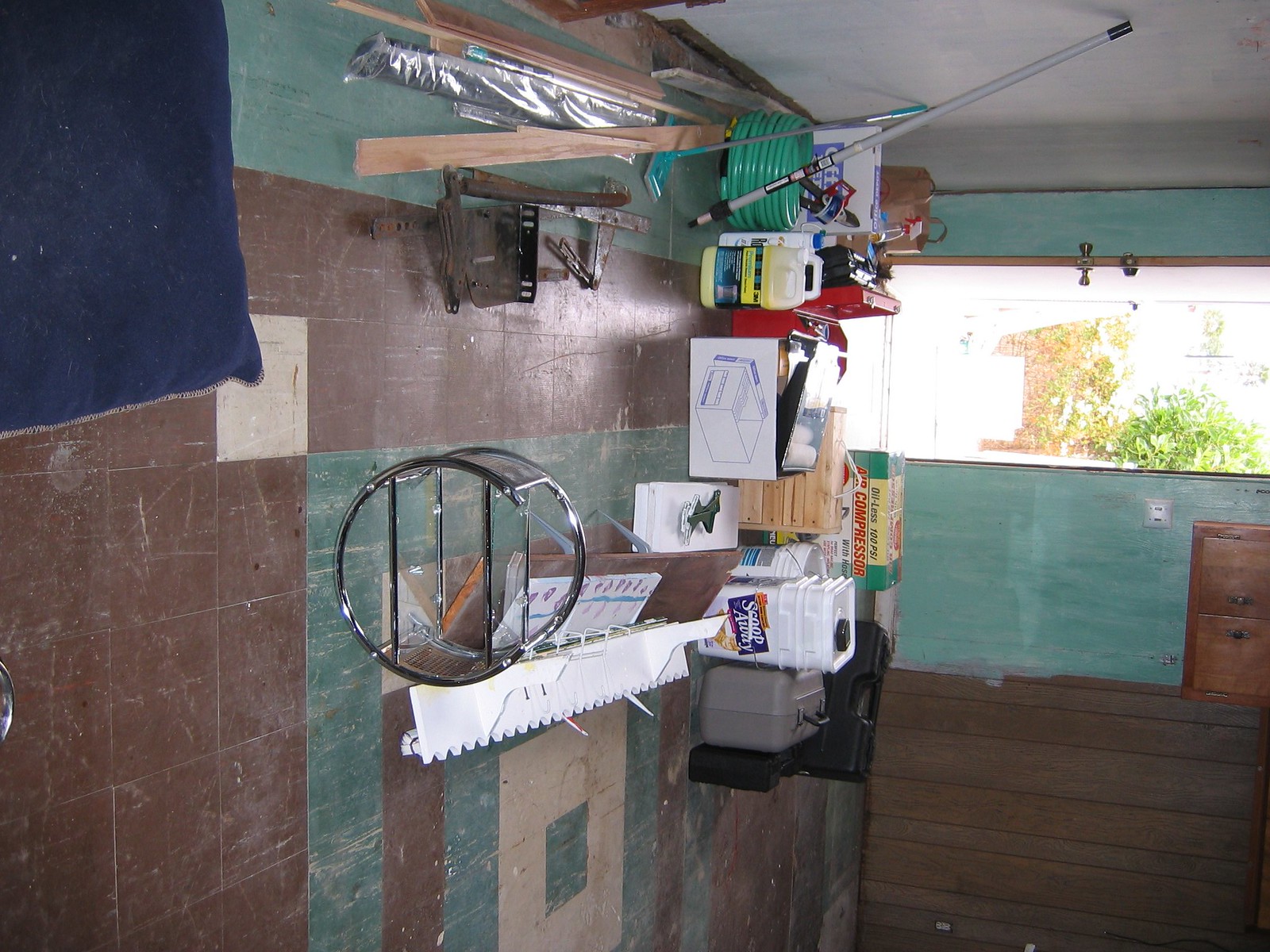The image captures a cluttered workshop or garage area, illuminated by daylight streaming through a small window on the right. Outside the window, patches of green grass and a hint of brown can be seen, though much of the view is obscured by an overabundance of white light. Inside, the walls are a mix of dark brown and sage green, both heavily scratched and appearing dirty, with white scratches and a smattering of tan and beige adding to the worn look. Various shelves are filled with an array of items: tool chests, a green water hose, wooden boards in the upper left corner, and a blue blanket hanging down. A silver circular object and a stack of white buckets are also visible, along with what appears to be a gray tackle box and a black briefcase, all contributing to the organized chaos of the space.